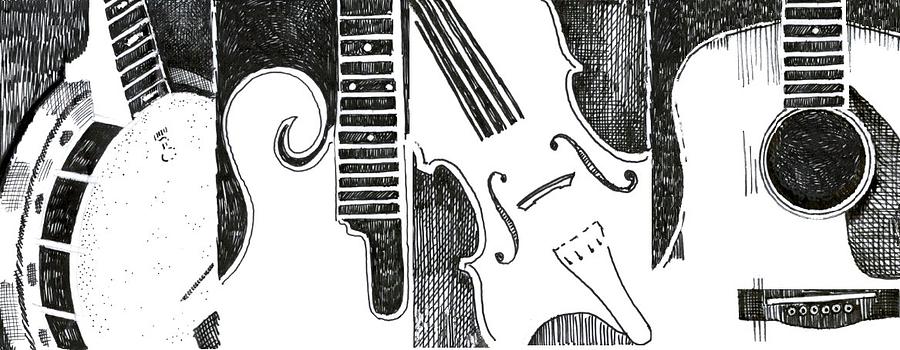The image consists of a detailed black-and-white compilation of four close-up line art illustrations of musical instruments, arranged from left to right in a landscape orientation. Each illustration focuses mainly on the body of the instrument with minimal visibility of the neck and is framed with intricate detail against a dark background. 

On the far left, the banjo is depicted with its circular body prominently shown, including the round drum top, partial metal rim, and a hint of the neck. Next is a guitar-like instrument, possibly an electric guitar or mandolin, distinguished by a unique curly-Q design near its neck. The third image features a violin, presented at an angle from top left to bottom right, highlighting its elegant curvature but offering no size context to infer whether it might be a cello. Finally, an acoustic guitar is depicted, showcasing its figure-eight shaped body, neck, and a hint of the pick guard. Each instrument is rendered in white against a predominantly black background, emphasizing the intricate line work and creating a cohesive visual harmony across the series.